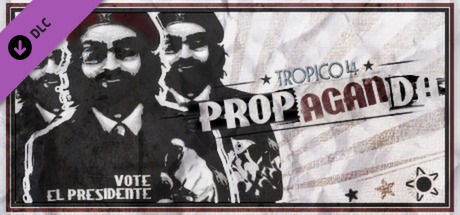This is a black and white poster, seemingly an ad for voting in a Spanish-speaking country. It features a horizontal rectangular design with three identical images of a bearded man wearing black sunglasses and a black three-piece suit. The man, who has longer hair and mustaches, is pointing directly at the viewer with his left hand. Beneath these images, the text "Vote El Presidente" is prominently displayed. In the top left corner, a purple strip, resembling a piece of cardboard, wraps around with the text "DLC" and a circle with a downward-pointing arrow. To the right of the images, the words "Tropico for Propaganda" are written, with some brown coloring in the text. The background includes rays of light emanating from the center, reminiscent of the Japanese flag design. At the bottom right, a black star, a red star, and a larger black star with a circle in the middle are featured, adding to the overall political campaign feel of the image.